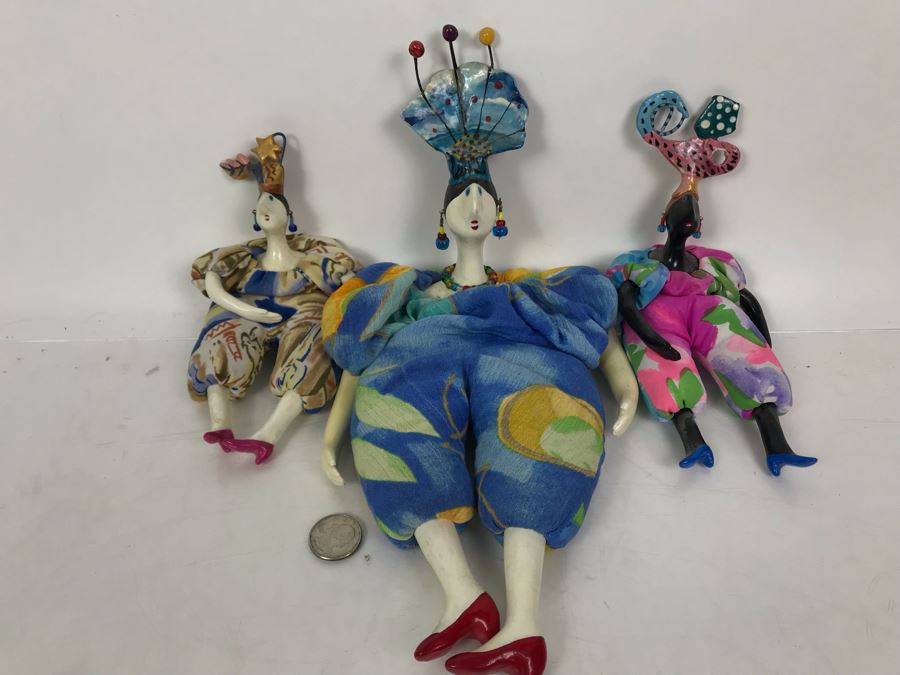In this indoor, horizontally oriented image, three dolls are leaning against a white wall with their bodies stretched out on the white surface in front of them. These dolls, with distinctly odd and almost alien features, are dressed in vivid, somewhat clownish attire, reminiscent of geisha or perhaps jesters, each with large, elaborate headdresses and colorful ensembles. The doll in the center, a white porcelain figure, is dressed in a predominantly blue outfit with red heels and white stockings, accented by a colorful headdress and a dime just below her right hand. To her right is a black-skinned doll donning an outfit in a mix of pink, orange, purple, and blue, paired with blue shoes and a matching headdress. The doll on the left, another white porcelain figure, sports a flashy cream-colored ensemble with accents of red, blue, and yellow, complemented by a similarly styled headdress and red shoes. A distinctive feature of this scene is a quarter placed on the ground near the central doll, adding a peculiar touch to the carefully detailed tableau.